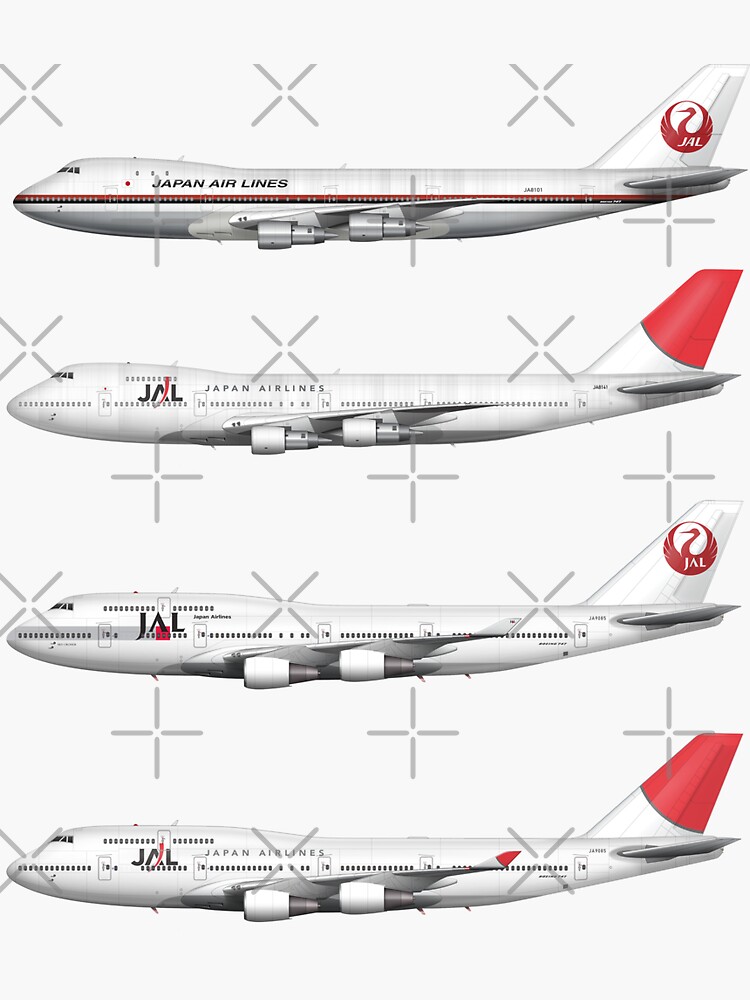The image depicts four Japan Airlines airplanes, flying horizontally, each showcasing distinct livery designs. All planes are predominantly white with black and red accents. The first airplane features the text "Japan Airlines" in black with a red and black strip running along the windows, and a circular emblem on the tail with "JAL" in white. The second plane has "Japan Airlines" in lighter dark writing and "JAL" in black on the front with a red strip on the 'A', and an all-red tail. The third aircraft has "JAL" in black block letters with a small red square under the 'A', no side strip, and a similar tail emblem as the first plane. The fourth plane mirrors the design of the second one, with "JAL" and the red strip through the 'A', red wingtips, and a red tail. The entire scene is set against a white background with noticeable watermarks running across in a pattern of X's and crosses.